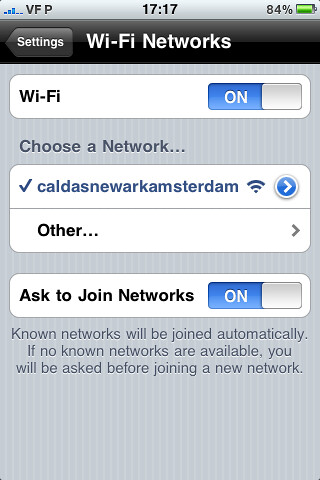The image is a vertical screenshot of a smartphone displaying the Wi-Fi settings page. At the top center of the screen, the time is shown as 17:17, flanked by "VFP" on the left and an 84% battery indicator on the right. The status bar also shows network signal bars. Below this, a green background is visible with a large black strip and a white settings button on the left side. The page title reads "Wi-Fi Networks." Underneath, a white horizontal strip indicates that Wi-Fi is turned on, highlighted in blue. Following this, the section titled "Choose a Network" lists the currently connected network, "Caldas, Newark, Amsterdam," marked with a checkmark and Wi-Fi icon. Other available networks are listed below this. The option "Ask to Join Networks" is enabled, as indicated by the blue switch. The informational text at the bottom states, "Known networks will be joined automatically. If no known networks are available, you will be asked before joining a new network." The overall screen background beyond these elements is gray.